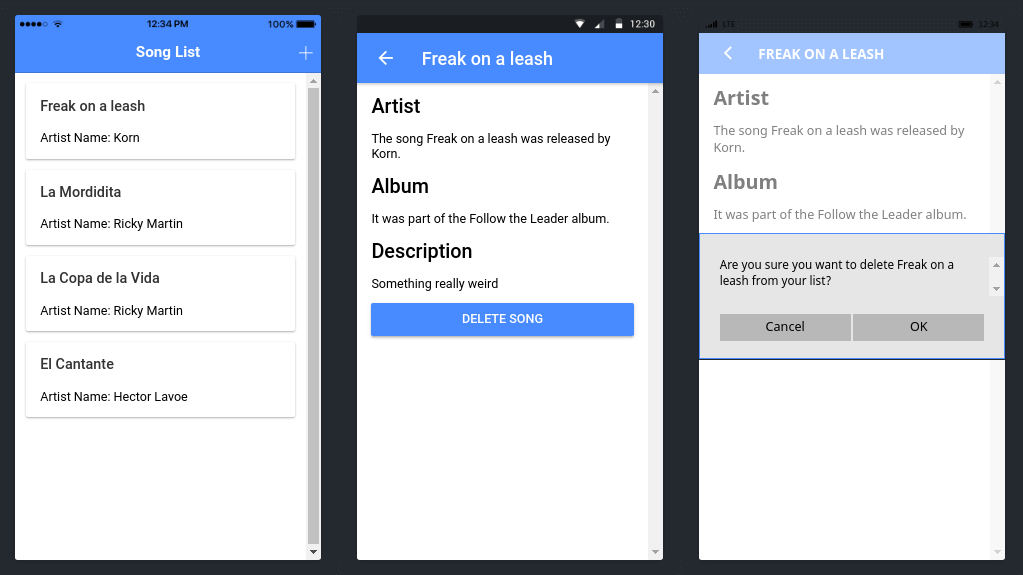This image showcases three separate screens, each featuring a blue-colored header at the top. On the leftmost screen, labeled "Song List," we see a detailed list of songs. The first entry is "Freak on a Leash" by Korn, followed by "La Mordida" by Ricky Martin, and another song by Ricky Martin subsequent to that. The next entry lists a song by Héctor Lavoe.

The center screen prominently displays detailed information about the song "Freak on a Leash" by Korn, including the album details. Below this information, there is a button allowing the user to delete the song from the list.

The rightmost screen reiterates the song "Freak on a Leash" and provides options concerning the song's management. It displays buttons that enable the user to either cancel or confirm the deletion of the song, along with the artists and album information.